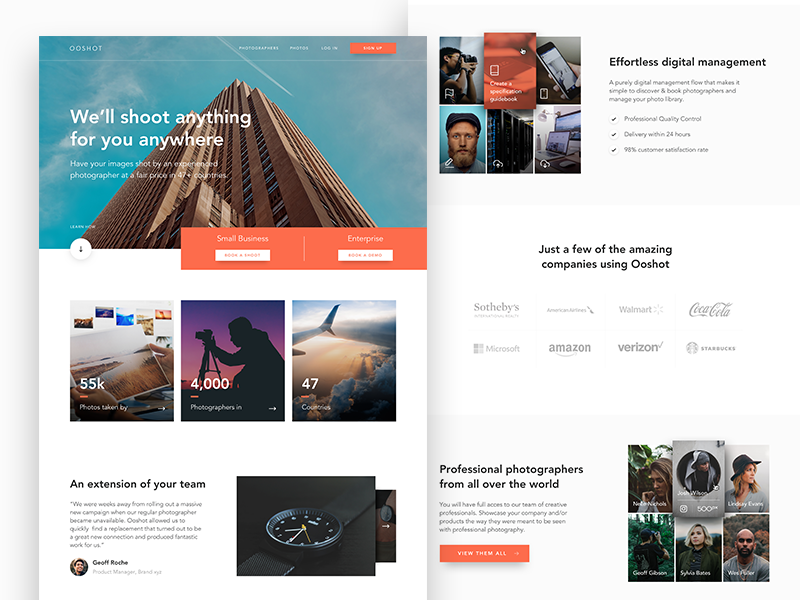This image is a screenshot of a web page featuring an advertisement for a digital management company. In the upper-left corner, there is very small text that appears to spell out "O-O-S-H-O-T." The advertisement seems to be spread across two pages.

On the left side of the advertisement, there is a striking photograph of a high-rise building against a clear blue sky. Below the photograph, an orange bar features two white clickable buttons, though the text on these buttons is unreadable.

The page includes several key sections with partially legible information. One section, titled "An Extension of Your Team," is accompanied by an image of a watch. Another section, labeled "Effortlessly Digital Management," is illustrated with a picture featuring a camera, an iPhone, and a laptop.

Further down, the text reads, "Professional Photographers from all over the world," which is supplemented by a series of six portrait photos showcasing diverse photographers. The text and images collectively emphasize the company's global reach and professional services in digital management and photography.